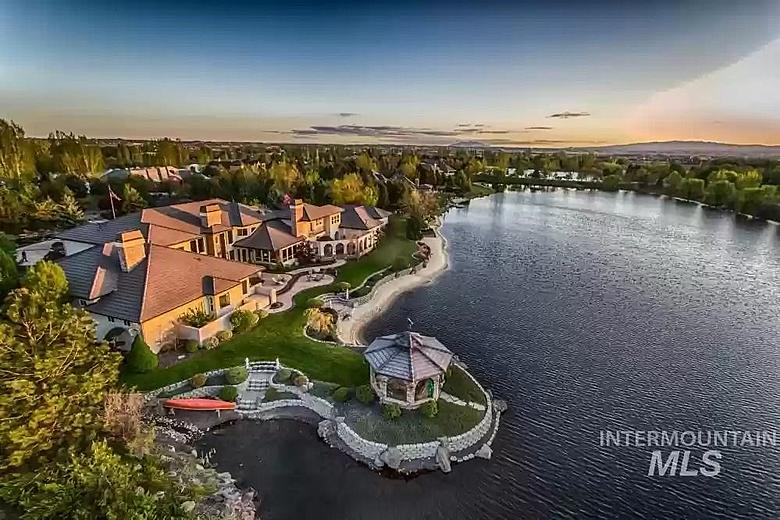This image provides an overhead view of an upscale lakeside property that exudes elegance. Dominating the foreground on the left-hand side is a sprawling mansion with a brown-tiled roof and a pristine white exterior. This grand structure features numerous windows and pointy roofs, reflecting a classic European architectural style. Adjacent to the mansion, closer to the center of the image, stands a smaller white building that could be a gazebo or a guest house. This building is designed with an octagonal shape and is topped with a round, gray roof adorned with a peak.

Stretching from the land into the shimmering blue lake, a dock extends invitingly into the water. The meticulously maintained green lawn around the mansion is dotted with lush trees, adding to the verdant scenery. In the backyard, a red boat is visible, enhancing the scene's charm. The backdrop reveals rolling green hills covered in dense vegetation and trees, adding a serene, rural touch to the setting, perfect for outdoor enthusiasts.

Additional houses and buildings are seen in the distance, suggesting the property sits in a desirable suburban or villa-like area. The water body, likely a lake or creek, wraps around the land, creating a picturesque scene with its reflective and sometimes choppy blue waters. The lower right-hand corner of the image contains text that reads "Intermountain MLS," which might indicate the location or provide some descriptive context for the property.